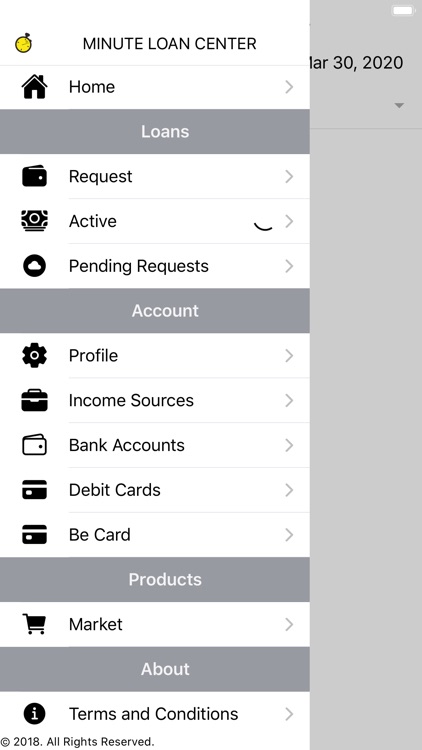This image, set against a white and gray background, depicts a detailed screenshot of a user interface for Minute Loan Center. At the top left corner, prominently displayed against a white background with dark gray text, is the title "Minute Loan Center" accompanied by a small clock logo to the left. Below this, there is a black home icon with the word "Home" next to it and a gray arrow pointing right.

Further down, there is a gray banner with the label "Loans" in white text, followed by a section with white background and dark text presenting several categories: "Request," "Active," and "Pending Requests." Another gray banner below these sections reads "Account" in white text. Under this banner, the interface lists several options from top to bottom: "Profile" (accompanied by a settings icon), "Income Sources," "Bank Accounts," "Debit Cards," and "B-Card," each with an arrow pointing right indicating further navigation.

Towards the bottom of the screenshot, yet another gray banner with "Products" in white text is visible. Beneath this, against a white background, there is a black shopping cart icon followed by the word "Market" in black text.